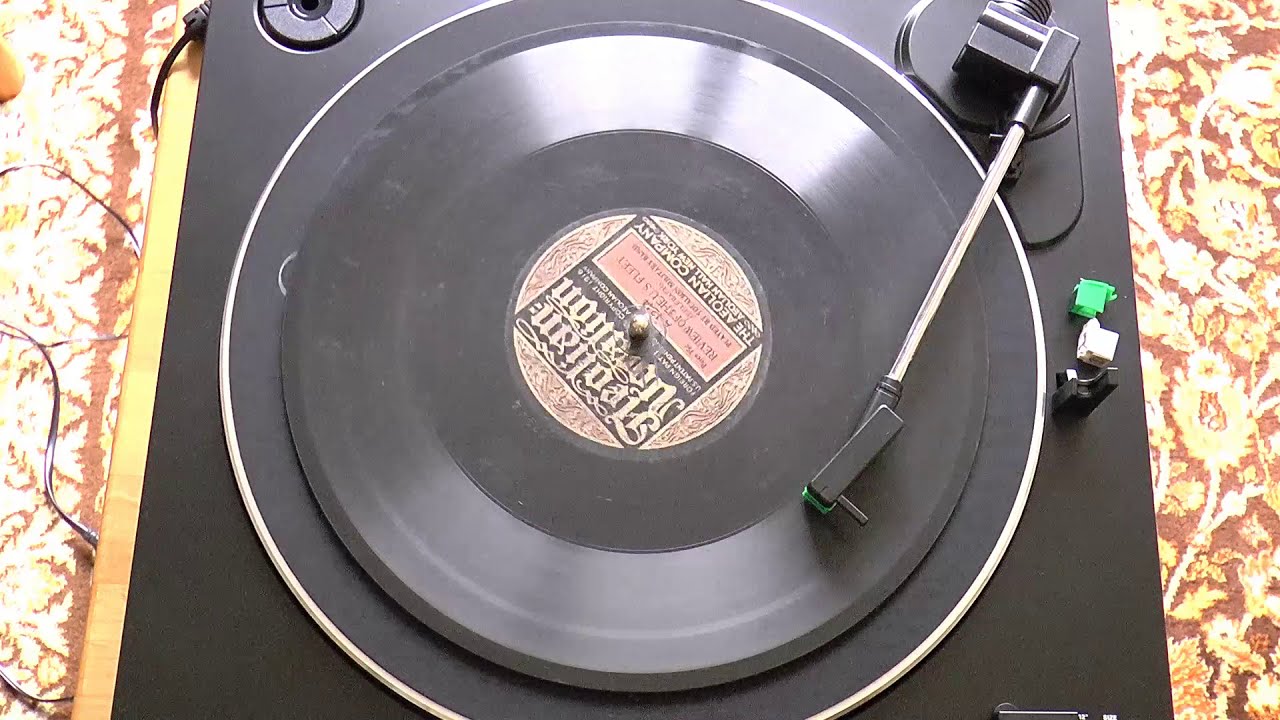The image displays a black, square-shaped record player positioned centrally on a red tablecloth adorned with a gold and white floral design. The camera provides a top-down view, revealing the needle engaged with a black record. The record exhibits a label featuring cursive text that is difficult to decipher, partially reading "A-E-O-U-I-A-N company," though this is not entirely clear due to its fancy font and upside-down orientation. On the right side of the record player, there are three small objects or needle covers in green, white, and black. The tablecloth, partly visible beneath the record player, enhances the vintage ambiance of the scene. Additionally, a wire extends from the left side of the record player, connecting it to an unseen device, suggesting that the record player is either paused or rotating slowly, as there is no visible motion blur on the record.